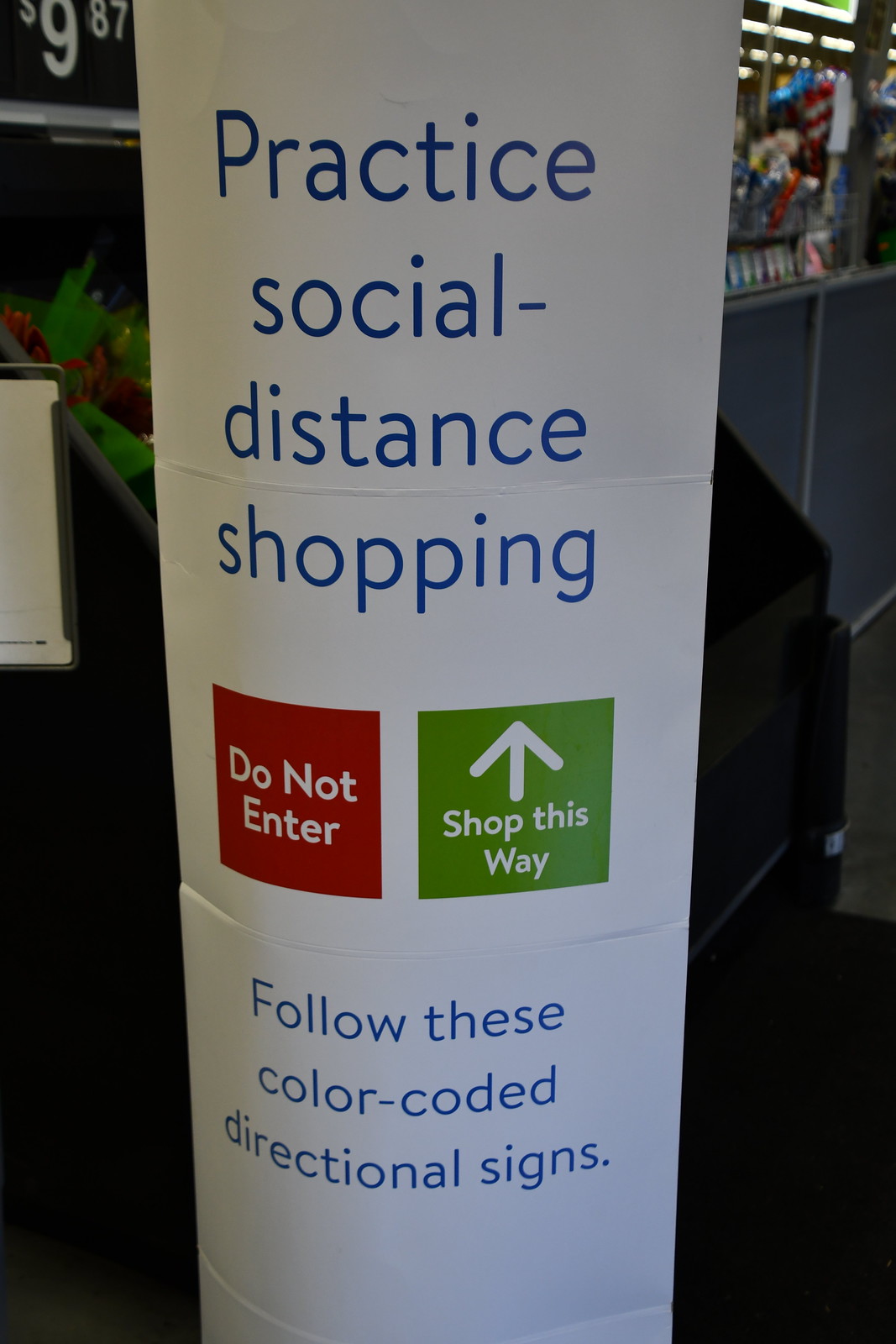The image depicts a white curved sign positioned outside a store, designed to guide customers on practicing social distancing while shopping. The sign features blue lettering and includes clear directives with color-coded boxes. A red box with white text instructs "Do Not Enter," while a green box with an arrow indicates the correct path with the message "Shop This Way." Additionally, the sign advises shoppers to follow these color-coded directional signs throughout the store. The backdrop of the scene includes a black cart filled with assorted flowers or green and red plants. In the upper right corner, there is a visible sign advertising a product on sale for $9.87. The windows behind the setup display more merchandise, giving a glimpse into the store’s offerings.